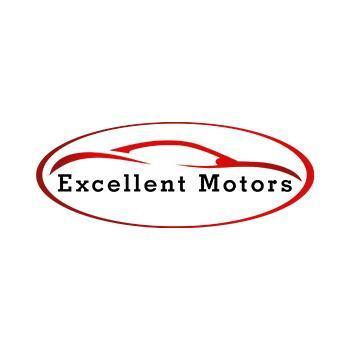The logo for Excellent Motors features a red, horizontally-oriented oval set against a white background. Within the oval, there are three red lines that curve to form the outline of a car's roof, evoking the sleek, aerodynamic shape of a vehicle. The first line is detached from the remaining two, which are interconnected. Below the curved lines, the text "Excellent Motors" is displayed in a bold, black font. The design elements create a striking contrast with the clean white background, highlighting the company’s focus on automotive excellence.